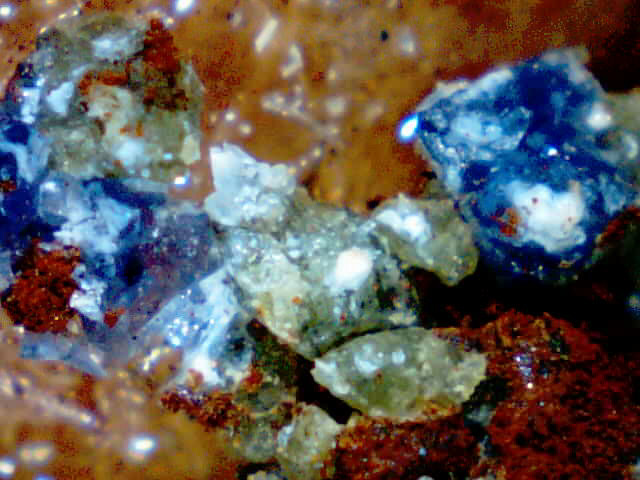The close-up image captures an unrefined and natural clustering of various crystals and stones, set against a backdrop of dark orange sand or gritty soil. Predominantly occupying the left to center-left region is a dark blue crystal, imperfect in shape but distinguished by white highlights and light blue accents, resembling a diamond. Scattered amidst these, particularly on the lower left, are clusters of light orange crystals, which also appear at the top left, hinting towards the center. The central part is characterized by semi-transparent, nearly clear crystals with a subtle greenish hue, interspersed with other clear crystals glistening under the light. In the upper right, another dark blue crystal with light blue accents complements the overall mosaic. Dominating the lower right quadrant is a substantial chunk of dark red crystal, completing the ensemble. This composition, strewn with specks of dirt and grit, vividly mirrors the untamed and raw splendor one might encounter while cave digging in nature.